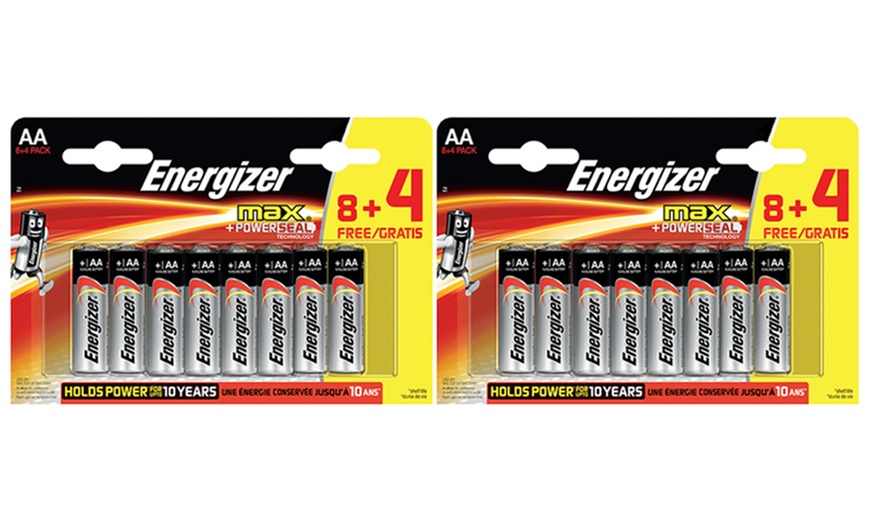In the picture, there are two identical packages of Energizer Max Plus AA batteries, placed side by side. Each package contains 8 AA batteries. The packages are prominently branded with the Energizer logo and feature a gray and black color scheme on the batteries themselves. 

The right section of each package is highlighted in yellow, and prominently displays the text "8 + 4 FREE/GRATIS," indicating a promotional offer of 4 additional batteries free with the purchase of 8. Additionally, there is a graphic icon of a person with a battery-shaped head on the packaging.